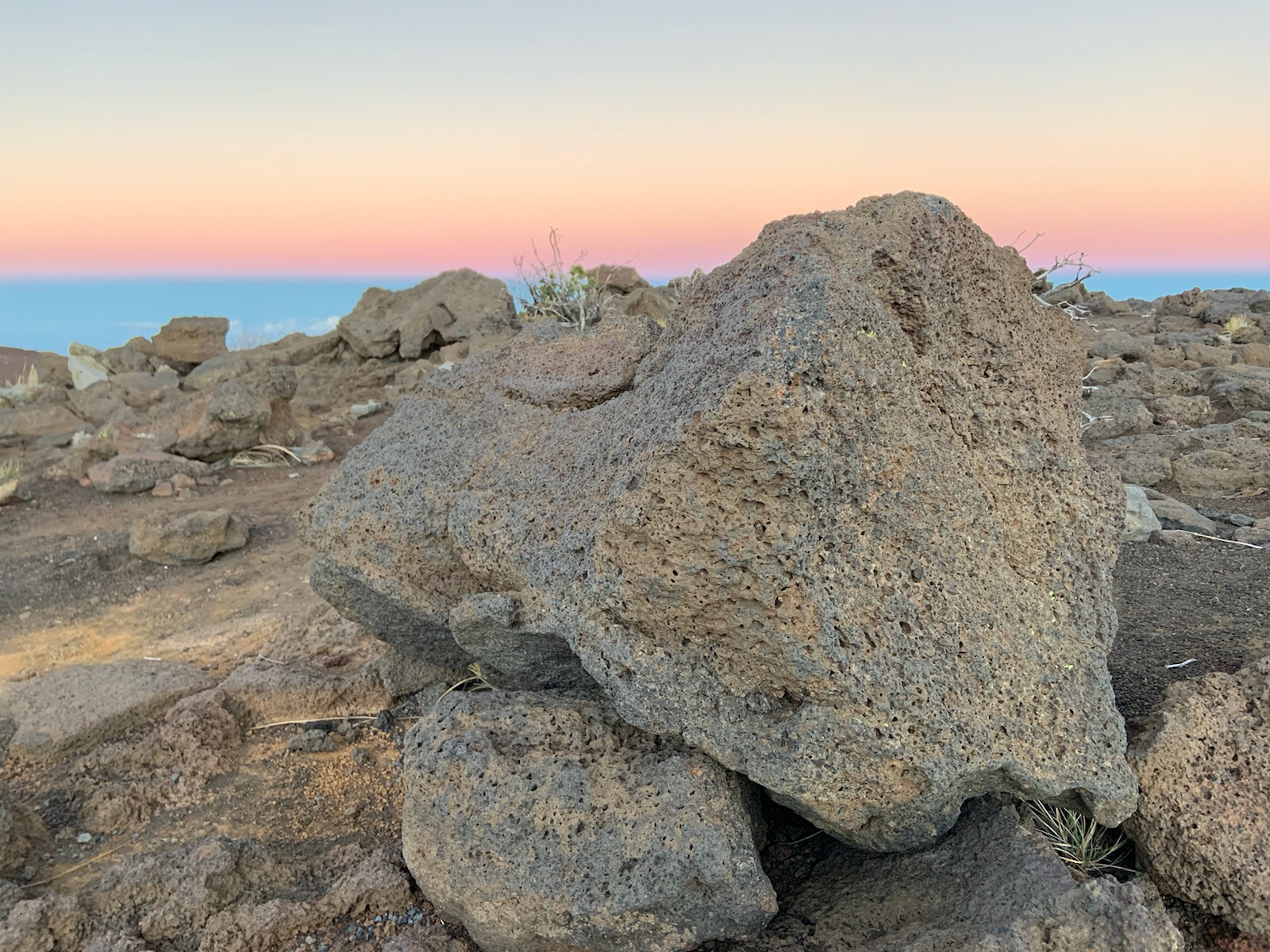The photograph captures an outdoor beach scene at sunset, showcasing a striking arrangement of light gray and tan rock formations with highly porous surfaces, resembling lava rock, covered in numerous pockmarks. Dominating the composition is a large boulder positioned atop several smaller rocks, with additional gray and brown rocks in the background. Wisps of dry, yellowish-tan grass sprout sporadically from crevices in the rocks. The sky transitions beautifully from a pale cotton candy blue near the horizon to vibrant shades of purple, red, orange, and yellow, culminating in a grayish-blue at the top. The image is devoid of animals, people, or text, allowing the natural elements and the vivid gradient of the sunset to take center stage. The clarity and focus suggest a professionally taken photograph, though some may find the subject matter itself understated.